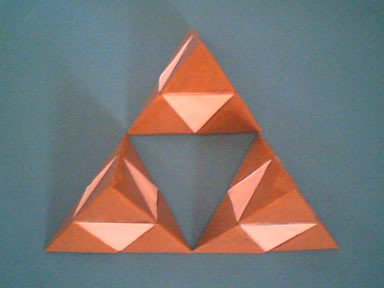The image depicts a geometric composition set against a light denim blue or turquoise background, transitioning from lighter in the top left to darker shades towards the bottom. The scene is lit from above, casting subtle shadows from the objects, enhancing the three-dimensional effect. Central to the image are three identical, three-dimensional pyramidal structures arranged in a triangle formation reminiscent of the Triforce from the Legend of Zelda. Each pyramid appears in a tan to orange hue and consists of smaller triangular segments: three orange triangles pointing outward from the center and a cream-colored triangle pointing inward, creating a cuboid illusion. This precise arrangement leaves a negative space at the center, forming another downward-facing turquoise triangle against the background. The meticulous placement and the interplay of light and shadow create a visually captivating and complex geometric pattern.